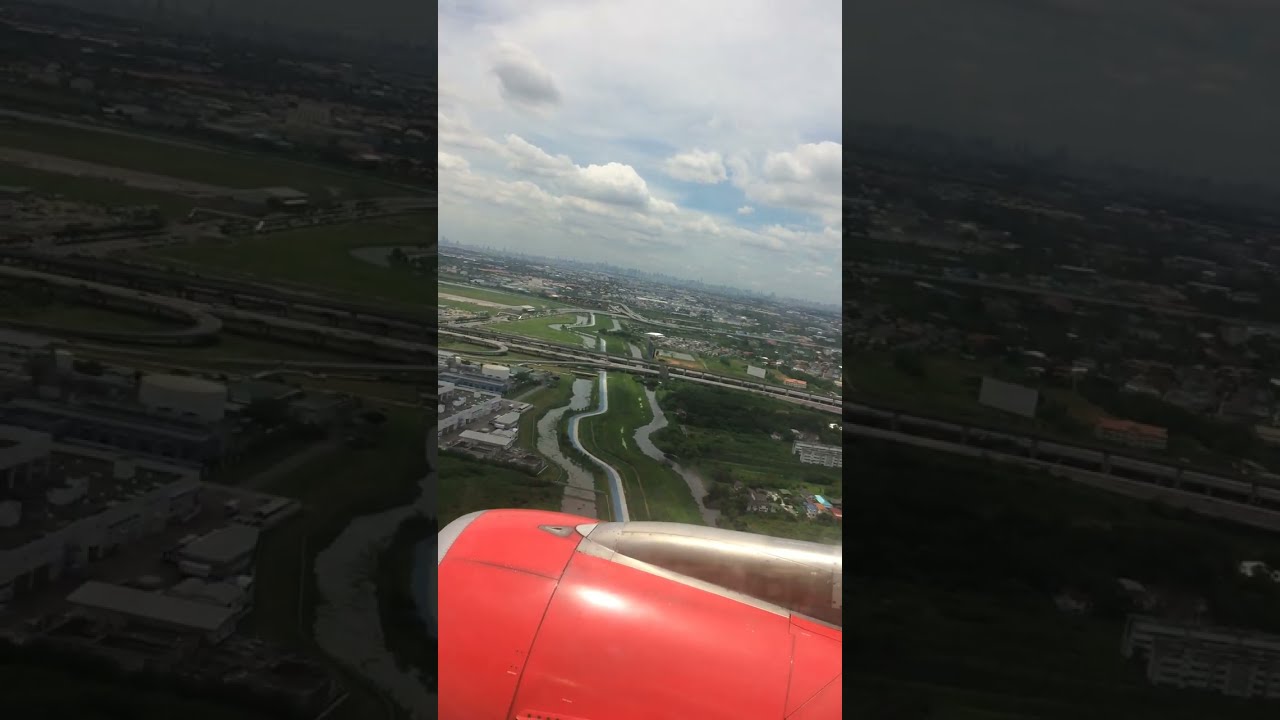The image is a vertically oriented, smartphone-style photograph taken from the window seat of a passenger airplane. The central view captures a red airplane engine cowling, showcasing its round propeller engine area with a silver vent on top, suggesting a jet engine type. Surrounding the aircraft, the sky is mostly blue with patches of gray clouds, creating a fairly cloudy day. Below, an aerial panorama reveals a cityscape with green grassy areas, tree-lined sections, and numerous buildings. Roads crisscross the landscape, and a prominent highway runs horizontally, intersecting with other paths. A bridge or roadway cuts perpendicularly across the scene. Additionally, tankers and urban structures near an airport are visible, emphasizing a flat land topography. The left and right portions of the image provide a zoomed-in continuation of this scene, enhancing the full scope of the landscape depicted from the airplane.